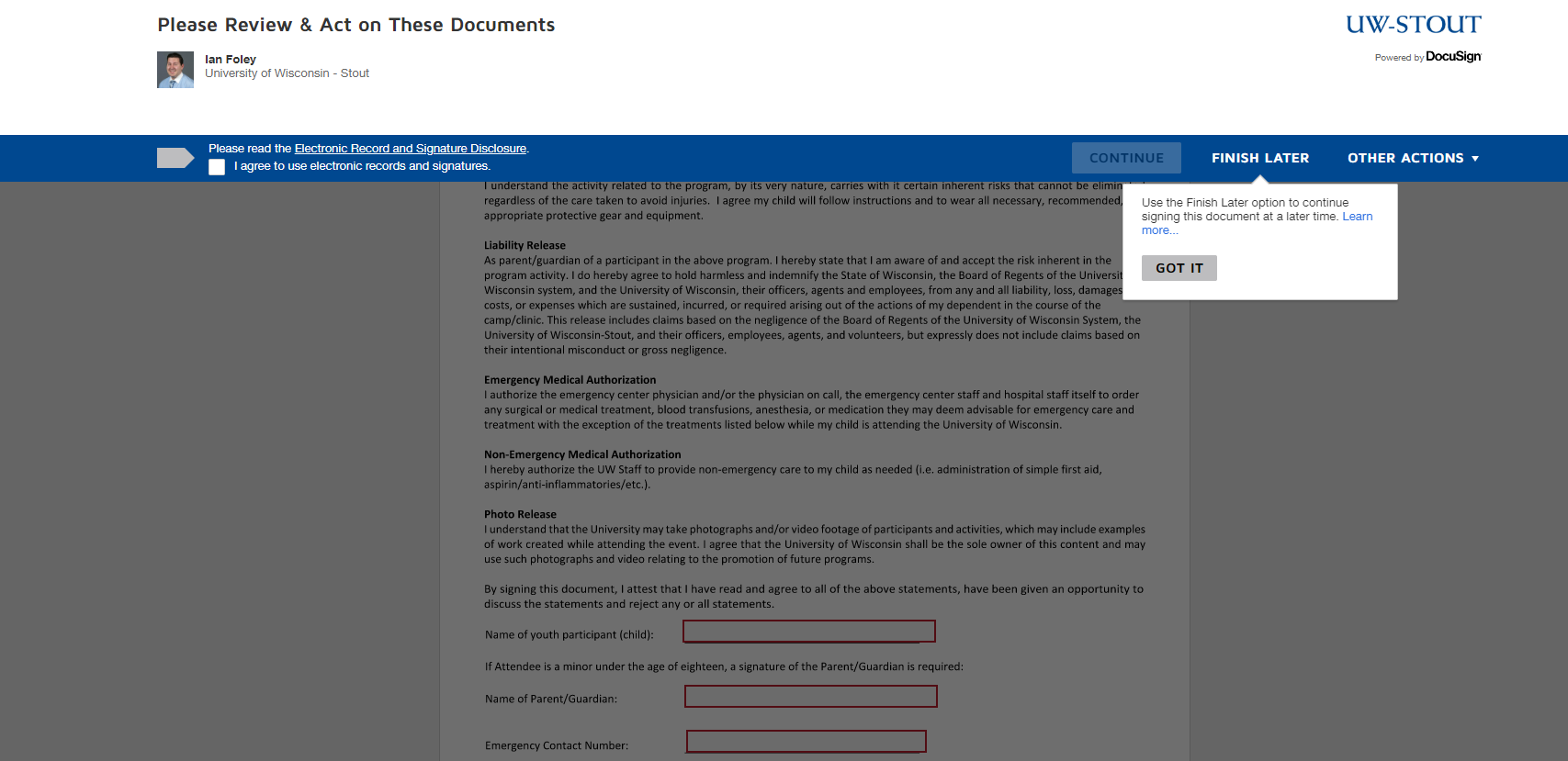The image displays a digital document with a white header that prominently features bold black text stating, "Please review and act on these documents." Below this header, centrally positioned, is a photograph of a Caucasian man wearing a light blue or light gray suit. The text beneath the photo identifies him as "Ian Foley, University of Wisconsin Stout." To the far right, an area is branded with the "UW-Stout powered by DocuSign" logo.

Just beneath Ian Foley's identification text, a dark blue section advises, "Please read the electronic record and signature disclosure." A gray arrow points toward an adjacent white checkbox that remains unchecked. Below this, aligned to the right, a button labeled "Continue" sits alongside a white "Finish Later" button.

An "Other Actions" dropdown menu appears under the "Finish Later" button. Expanding from this menu, a white rectangular tooltip informs users, "Use the Finish Later option to continue signing the document at a later time." Within this tooltip, a "Learn More" hyperlink is present, and directly below, a gray "Got It" button provides an option to acknowledge the message.